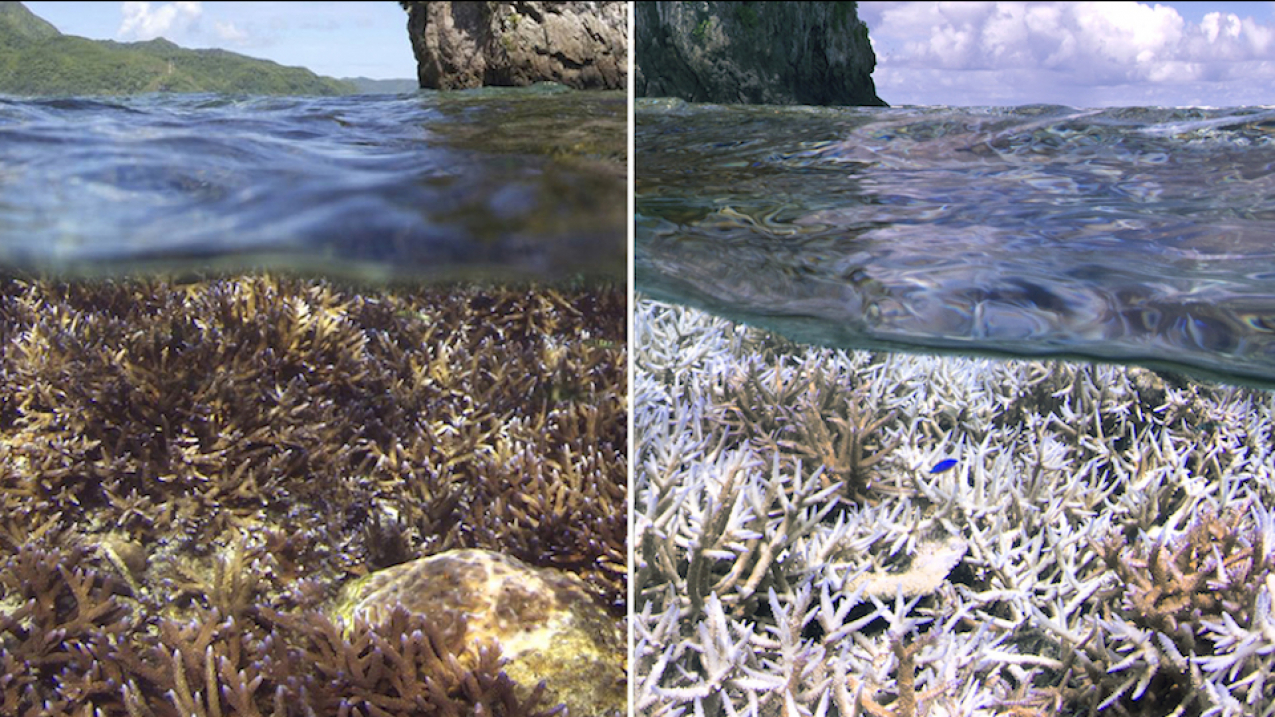This side-by-side photograph captures two underwater scenes taken at the same location, just on opposite sides of a giant rock protruding from the ocean. The image, taken with a half-submerged camera, displays a striking contrast between the two sections both above and below the waterline.

In the left photo, the above-water scene showcases a majestic mountain range, partly covered in rocks and vegetation, set against a clear blue sky adorned with wispy white clouds. A portion of the giant rock that juts out of the ocean is visible in the upper right corner. Below the waterline, a vibrant underwater world is revealed, with a seafloor teeming with brownish and orangish corals and sea plants, indicating a healthy, flourishing marine environment.

Conversely, the right photo presents the above-water view of the same rock formation, backdropped by a sky filled with big, puffy clouds. Below the waterline, the stark difference is evident as the corals and sea plants appear bleached and white, contrasting sharply with the thriving underwater flora seen in the left photo. This side also features a tiny blue fish swimming in the center, adding a splash of color to the otherwise bleached underwater landscape. The ocean surface appears calm in both images, captured on a seemingly bright, sunny day. Together, the photos may indicate an environmental before-and-after scenario, highlighting the impact on marine life across different sections of the same location.